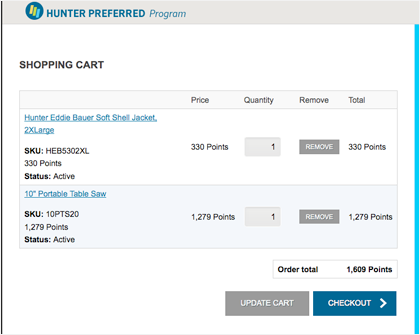Screenshot of a Hunter Preferred Program shopping cart showcasing two items. The first item listed is a Hunter Eddie Bauer Softshell Jacket, priced at 330 points, with a "Remove" button next to it. The jacket's SKU is HEB 5302XL, and its status is "Active." The second item is a 10-inch Portable Table Saw, priced at 1,279 points, also featuring a "Remove" button. Its SKU is displayed, and the status is marked as "Active." The subtotal for the two items is marked as 1,609 points. Additionally, the cart has an "Update Cart" button and a "Checkout" button. The interface mainly includes functionalities for adjusting the quantity of items and proceeding with the purchase. Based on the item descriptions and overall theme, the site appears to be related to hunting or outdoor activities.